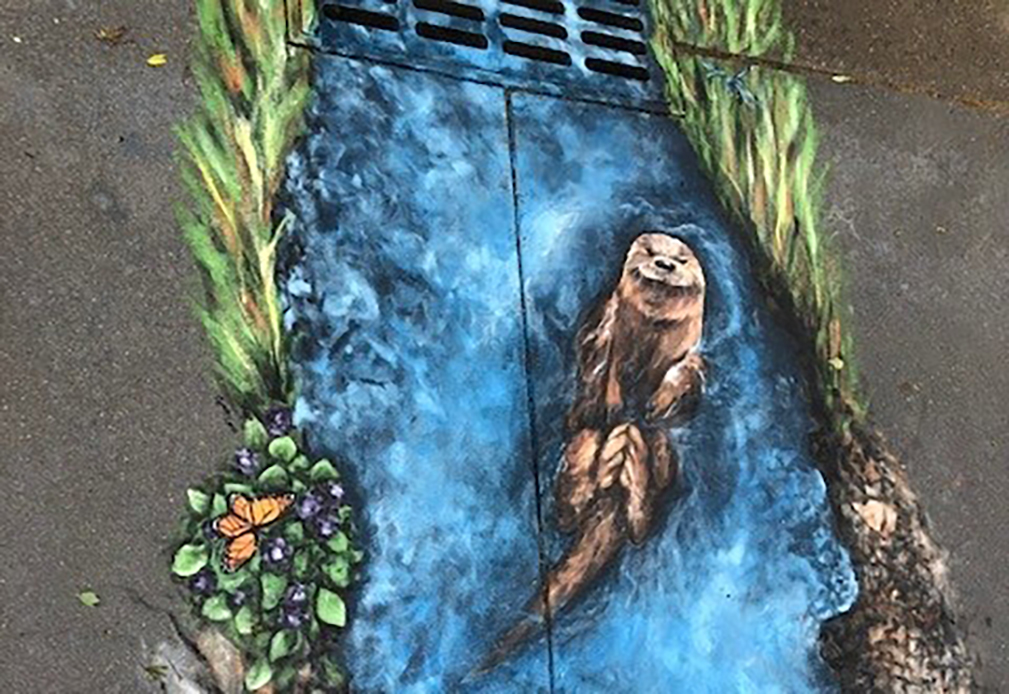The image shows a detailed, painted mural on the ground, depicting a vibrant blue river flowing along a dirty concrete surface. The center of the mural features a light brown sea otter with a long tail and a facial expression that appears to be smiling upwards. The otter is floating on its back in the river, with its limbs folded close to its body. Surrounding the river on both sides are grassy green banks, enhancing the natural scenery. On the bottom left corner, there is a purple-flowered bush with an orange monarch butterfly perched on it. The top of the mural includes a storm drain or grate, giving the illusion of the river flowing into it. The painted landscape contrasts with the real unpaved dirt visible in the top right corner and scattered bits of leaves and dirt across the entire scene.